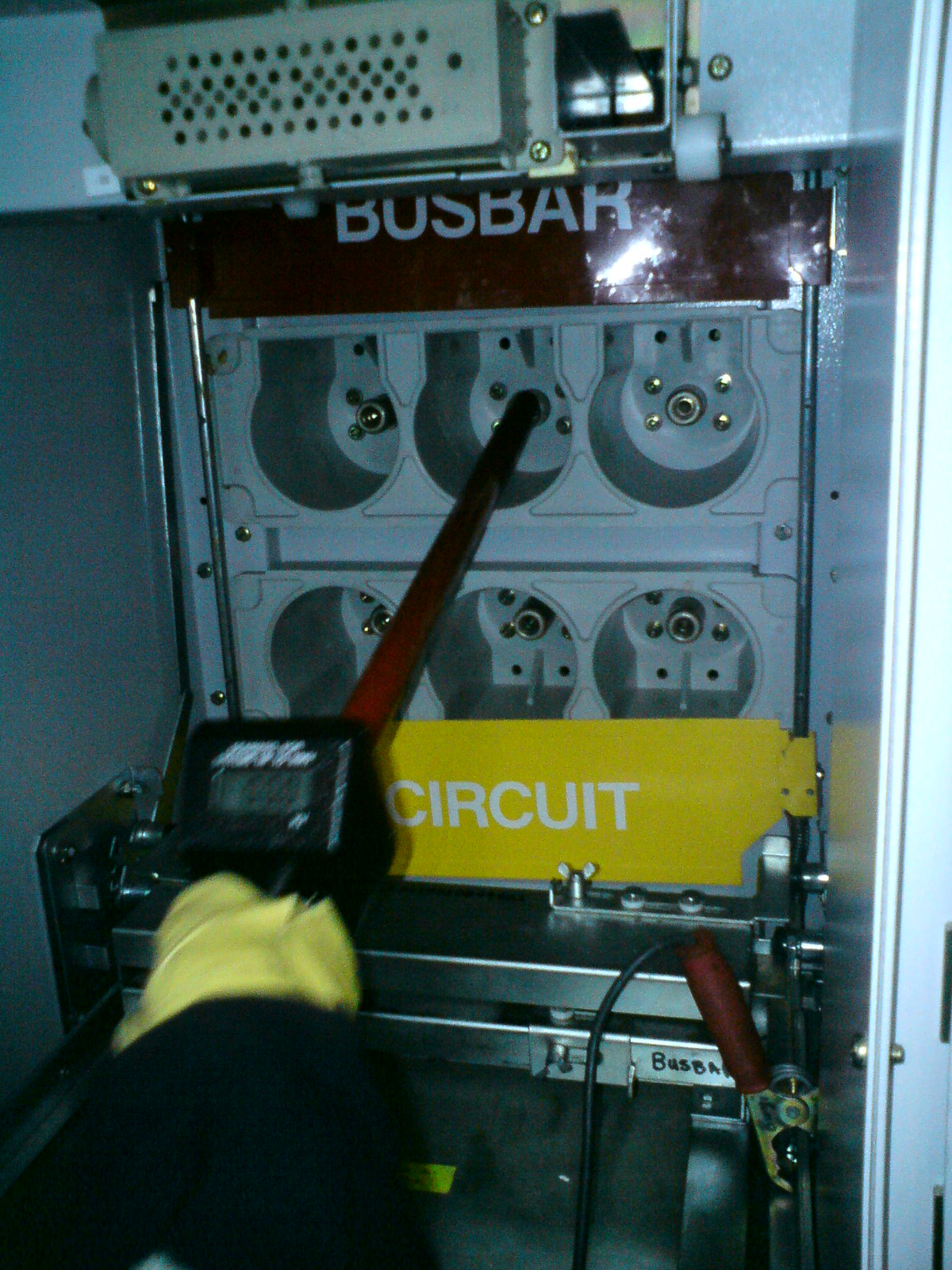In the photograph, a person's arm, clad in a yellow glove, is seen holding a sophisticated piece of testing equipment. The device, a black cubic meter with a digital readout screen showing "000" in black text on a gray background, is held steady. Above the screen, some white text is present but is blurry and unreadable. Emerging from the top of the meter is a long red cylindrical rod. This rod is being carefully inserted into a hole on the side of a metallic gray piece of equipment. The equipment features two rows of three holes each, with the rod inserted into the top row's middle hole. Above these rows is a red horizontal sign with "Bus Bar" written in white. Below the holes, there's a yellow sign with "Circuit" also in white letters. Nestled in the bottom right corner of the image, a red jumper cable with a yellow-tipped clamp and a black wire can be seen. The overall setup appears to be part of an intricate electrical testing or circuit-breaking procedure.